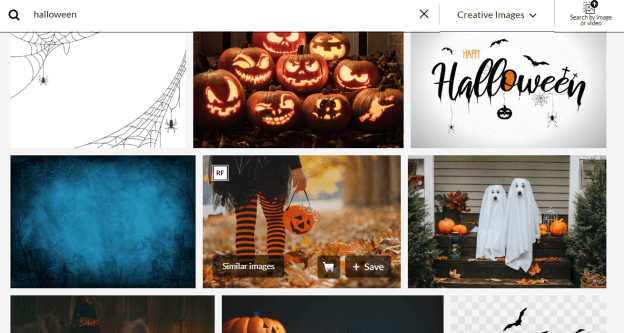The top left corner of the image features a black search bar icon followed by the word "Halloween." Adjacent to it is the label "creative images" with a drop-down arrow, and next to that, there is an option labeled "search by image or video," which allows users to upload their own images or videos for searching. 

Beneath this search bar are a series of squares populated with Halloween-themed visuals. The first square displays a white background with two spiderwebs; one web is located in the bottom right corner while another is at the top left corner, each hosting a hanging spider. 

The second square showcases a stack of carved pumpkins with candles placed inside to illuminate their various facial expressions.

The third square features the word "Halloween" written in cursive with bats flying in the background, adding to the spooky theme.

The final square presents a light blue forest background, providing a serene yet slightly eerie atmosphere.